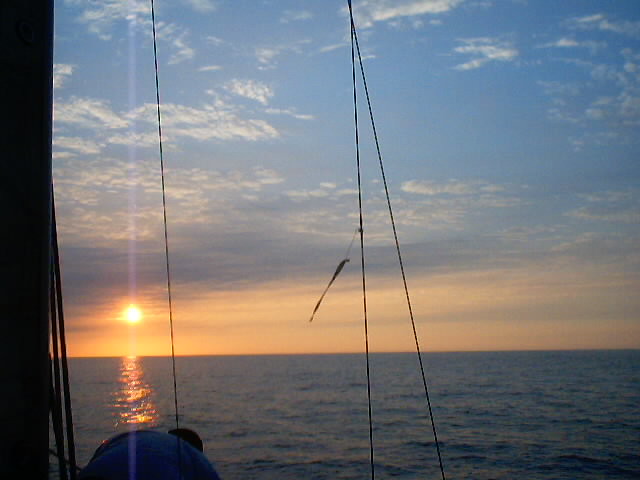The image captures a serene scene of the ocean during either sunrise or sunset. A man, wearing a blue shirt and possibly a mask, is seen bending over on what appears to be a sailboat, inferred from the presence of several strings or lines that extend from the bottom to the top of the image, suggesting rigging. The boats' specific parts are not visible, but a dark shadow, likely a mast, occupies the far left edge of the image, reinforcing the setting as on a ship or sailboat. The lower quarter of the image shows the tranquil sea, while the upper three-quarters magnificently display a blue sky adorned with small, white, wispy clouds. The sun is hovering just above the horizon in the lower left corner, contributing to the breathtaking colors and ambience of the sky and sea.